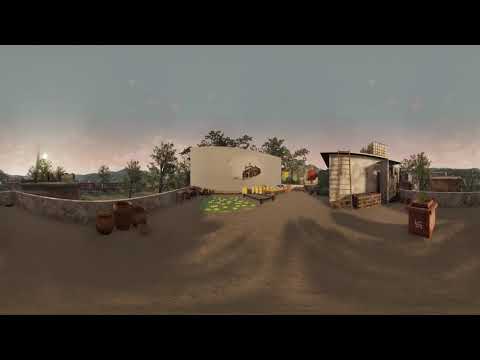The scene appears to be an outdoor, computer-generated environment, likely from a game, with a soft and slightly stylized quality to the graphics. In the foreground, there is a sandy or dirt-covered path. On the left, a stone wall extends into the distance and meets a series of barrels, leading towards a central structure. To the right of this structure is a small rectangular building with a gray-tan exterior, featuring a wooden ladder resting against its side. Adjacent to this building is a white concrete structure with an additional ladder extending up to its roof. Mirrored on the right side is another continuation of the stone wall, which frames the scene.

In front of the buildings and structures are various objects, including cylindrical containers and a rectangular plastic trash can, lending to the environment's lived-in feel. Scattered around are some smaller wooden boxes. Surrounding this central area is a backdrop of trees, providing a natural barrier, with more trees placed selectively in the foreground. Further beyond the trees, a range of mountains stretches across the horizon from left to right, enhancing the scenic panorama. Above this mountainous backdrop is a bluish-gray sky, tinged with pink near the bottom, suggesting the sun is setting or has just set, as indicated by the warm light and lack of clouds. This scene captures a tranquil yet detailed moment at dusk, blending elements of nature and man-made structures seamlessly.